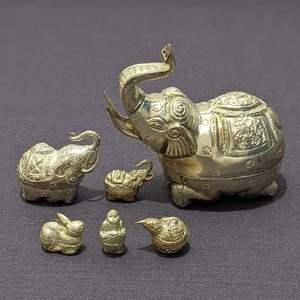This image is a color photograph showcasing six meticulously crafted figurines arranged on a textured gray fabric backdrop. The figurines, which appear to be carved from a light tan or grayish material, potentially cast, vary in size and represent different animals.

In the back row, there are three elephants, each adorned with intricate, ornate designs. The largest of these, located on the far right, faces to the left and features an elaborate saddle on its back. To its left is a medium-sized elephant, also facing to the right, with similarly detailed embellishments around its ears and head. The smallest elephant, situated furthest to the left, mirrors the medium-sized one in design and direction.

In the front row, the figures depict a range of animals carved from the same material. On the far left is a rabbit, positioned to face the right. The central figure is a monkey with a forward-facing posture, though it could be mistaken for a man due to its small size and ambiguous features. The rightmost figure in the front row is a chubby bird with a round body and elongated beak, resembling a kiwi bird, facing towards the left.

This collection of intricately designed figurines, each unique in size and detail, forms a charming and visually appealing ensemble.